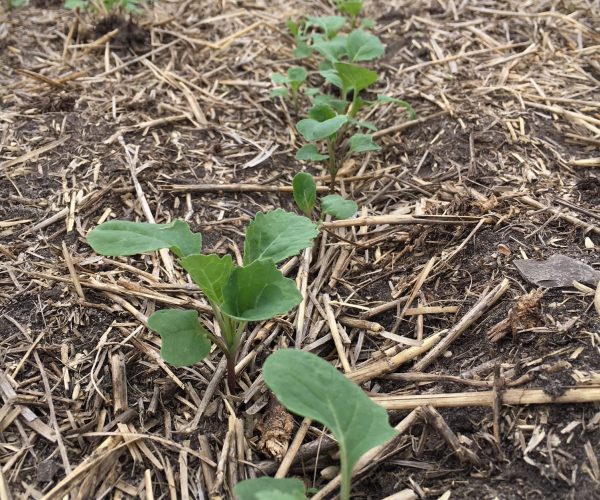This outdoor photograph captures a ground area where a row of small green plants with oval-shaped leaves, approximately four inches tall, is sprouting from black soil. The soil surface is scattered with light brown, dried twigs and straw, giving a yellowish-brown tinge to the scene. The plants, which might be crops or possibly weeds, are emerging through the straw, which appears to be randomly dispersed across the rectangular frame. The overall scene exudes a natural yet cultivated feel with the vibrant green plants contrasting against the dry, muted tones of the surrounding twigs and straw.